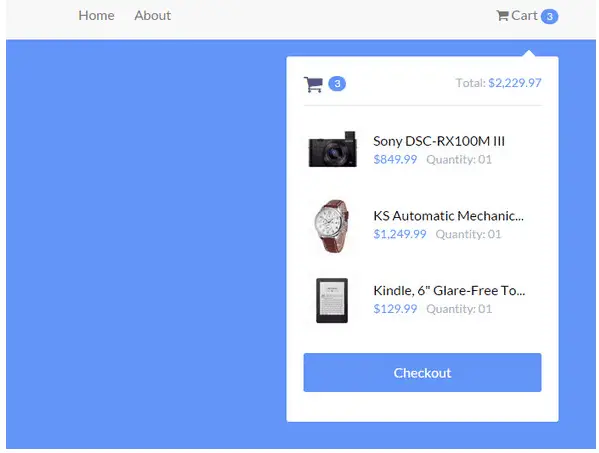This image appears to be a detailed screenshot of a shopping cart section from an e-commerce website. The image is square-shaped and features several distinct areas:

At the very top, there's a narrow, light gray horizontal bar that spans the entire width of the image. Near the top left, slightly off-center, there are clickable text options in black: "Home" and "About," likely leading to the homepage and an information page about the company or website respectively. 

In the top right corner of this gray bar, there's a black cart icon next to the word "Cart," accompanied by a blue circle containing the white number "3," indicating three items in the cart.

The main background of the image is predominantly a pleasing shade of blue. Centrally focused is a white vertical rectangular section representing the cart's content. This section has a small triangular pointer at the top, directed towards the cart icon, emphasizing that we are viewing the cart contents.

Within the white rectangular section, there's a repetition of the cart icon and the blue circle with the number "3" at the top left. To the right, the word "Total" is presented in gray, followed by the total amount of $2,229.97 in bold blue text. 

Below the total, the three cart items are listed one below the other. The first item is a camera with an accompanying image labeled "Sony DSC-RX100M3," priced at $849.99, quantity one. The second item is a watch with a white face and a brown leather band, labeled "KS Automatic Mechanic," priced at $1,249.99, quantity one. The third item is a black Kindle with a white screen displaying text, labeled "Kindle 6-inch glare-free," and priced at $129.99, quantity one.

At the very bottom of the white section is a blue rectangular button with the white text "Check Out," inviting the user to proceed with their purchase.